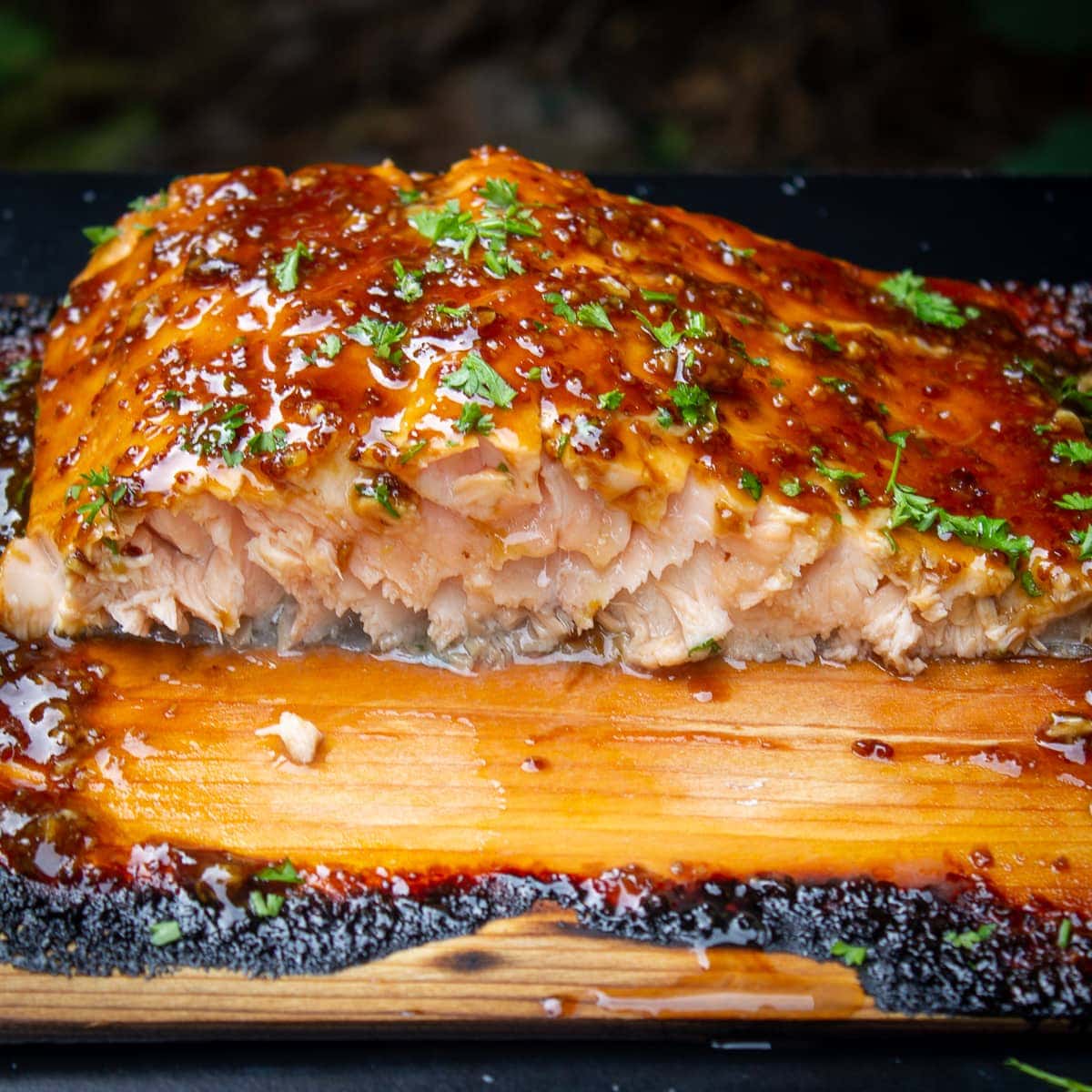This close-up photograph captures a delectable, partially cut piece of grilled salmon on a rustic wooden cutting board. The salmon, showcasing a light pink interior, is adorned with a beautifully caramelized brown glaze, giving it an appetizing sheen. The surface is sprinkled with fresh, green parsley and other subtle seasonings, enhancing its visual and flavorful appeal. The cutting board exhibits some charred areas, indicative of the grilling process, adding to the rustic charm of the setting. The blurred background hints at an outdoor environment with hints of a black table and green foliage, further emphasizing the freshness associated with the dish. This meticulously prepared and presented salmon looks incredibly delicious, ready to be enjoyed.